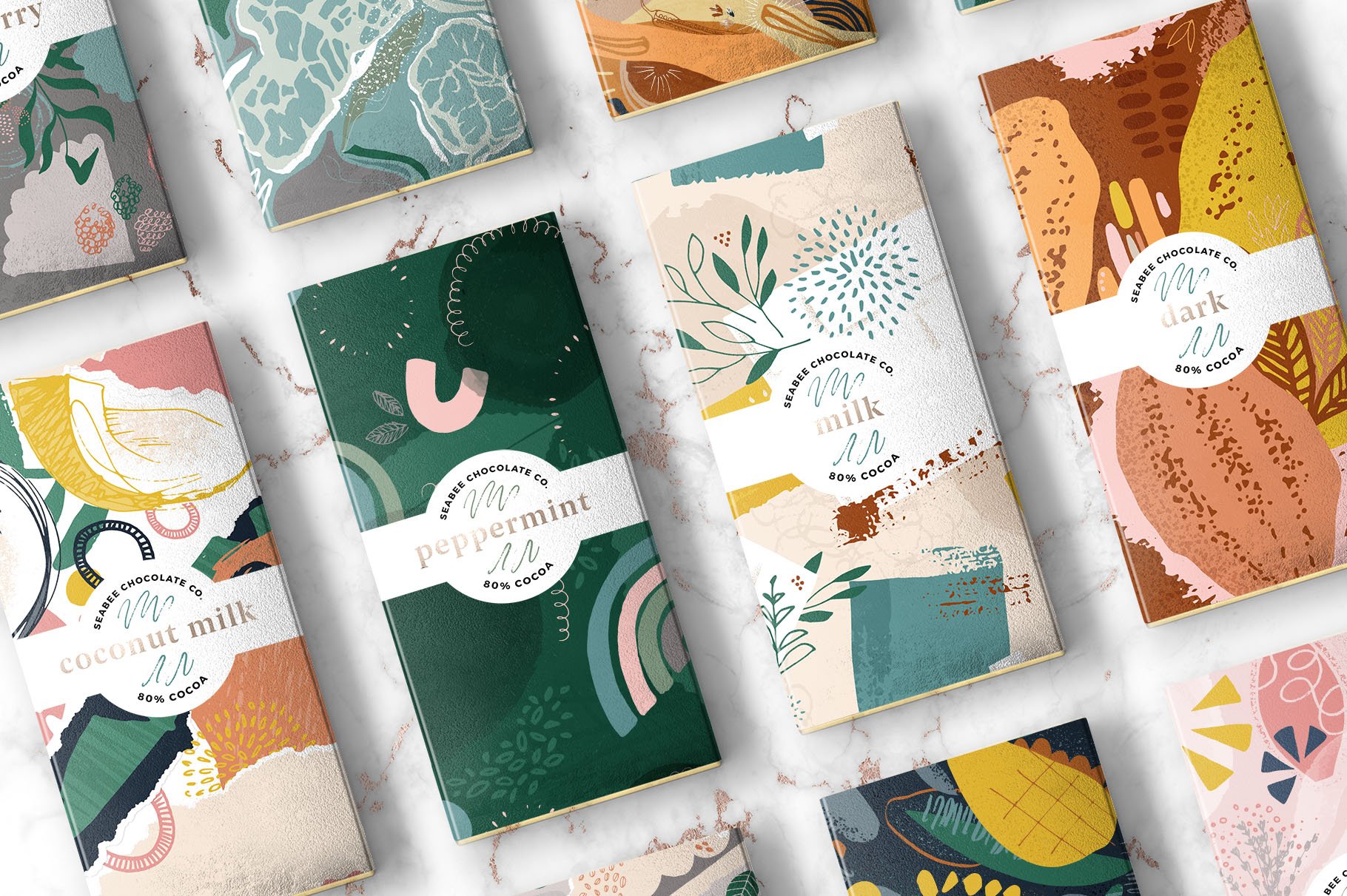The image depicts a variety box of chocolates from the Clever Chocolate Company, featuring four distinct flavors, each labeled and uniquely packaged. From left to right, the flavors are: Coconut Milk, enclosed in a colorful package with hues of pink, orange, green, and white; Peppermint, wrapped in a green package; Milk, set against a beige backdrop with leaf designs and labeled with the words "Bond Cocoa"; and Dark Chocolate, encased in a package with rusty orange and yellow tones. The overall design of the box includes thin white and gray borders between each chocolate flavor, giving it a segmented, organized appearance. The chocolates boast 80% cocoa content and are encased within a packaging that resembles a grid or barred structure. There are a total of 12 different flavors, although only four are visible. The branding prominently displays "CCSEASE" at the top.